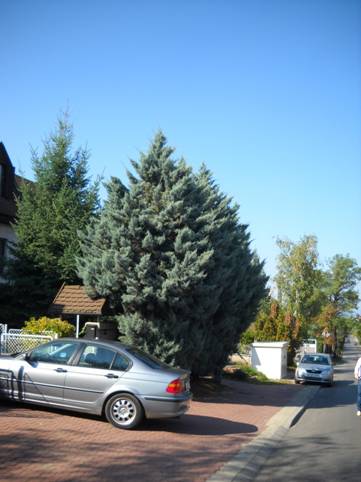The image captures a vibrant, well-kept residential street on a sunny, cloudless day. Dominated by a vast expanse of blue sky, it features an abundance of lush trees, mostly pine, with a few hardwoods mixed in, especially on the right side. The landscape is meticulously maintained, with beautiful greenery and a red brick-paved driveway adding to its charm. 

In the foreground, a gray four-door sedan is parked in the driveway, in front of a chain link gate and a structure with a brown roof. Another car, silver in color, is somewhat propped up on the curb, facing the viewer from the right side. Partially visible on the lower right is a person in jeans and a long white shirt, possibly taking a walk. The composition illustrates a tranquil, picturesque neighborhood with neatly arranged elements and vibrant natural light.